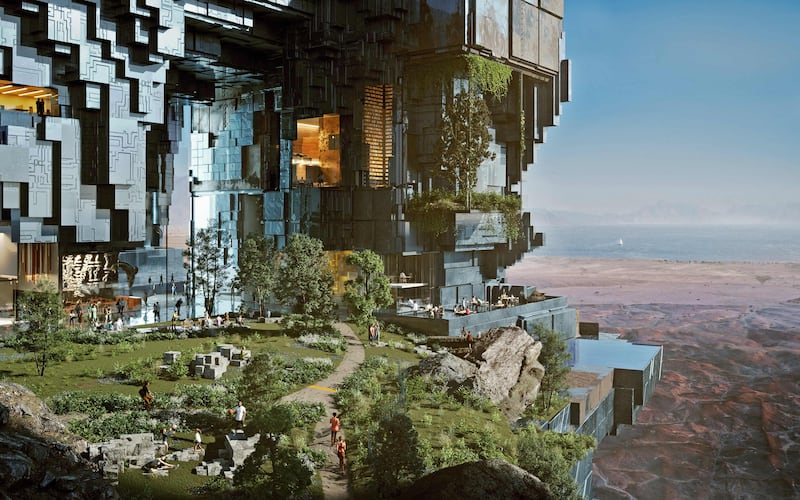This rectangular, landscape-oriented digital illustration depicts a futuristic cityscape with a prominent, gargantuan, modern-looking building on the left half of the image. The structure is characterized by dark, blocky, geometric shapes—squares and rectangles—that jut out and descend along a cliffside. Integrated into the building are numerous terraces with lush grass and trees, adding green patches to the stark, modern design. One notable feature is a large arch that extends off to the left.

In the lower left corner, there is a park-like setting with walkways, trees, and abundant grass. People are seen walking, playing, and riding bikes in this tranquil area. Further to the right, on one of the building's overhangs, there are tables and chairs where diners are seated, enjoying the view.

The right one-third of the illustration presents a stark contrast, depicting a barren valley with shades of brown, featuring rugged, hilly areas. Beyond this valley, a blue sky stretches above a waterline that is barely visible in the distance, framing the tranquil yet desolate background. This combination of elements creates a visually striking scene that juxtaposes futuristic architecture with natural landscapes.